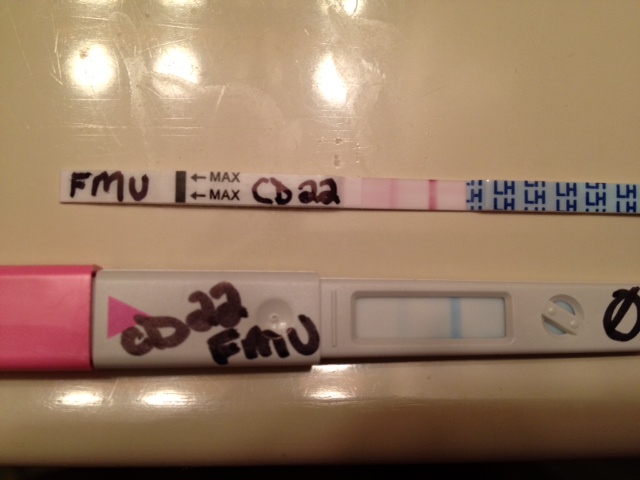The image is a close-up of a coral thermometer with intricate detailing. The thermometer features a distinct pink cap on the left end, transitioning to an off-white body. Next to the pink cap, there is a black marker inscription reading "CD22FMU". Adjacent to this marker is a reader screen displaying a blue vertical line slightly right of center. 

Further along, there's a circular design element followed by a marker indicating zero, crossed by a line. Above these is a control strip, appearing as a thin, elongated piece of paper. At the top of the strip, the label "FMU" is prominently visible. Below this, a black horizontal line is labeled "max" twice, accompanied by two arrows pointing to the right. 

Next to these markers, the inscription "CD22" is present alongside a prominent red line, somewhat right of center. At the bottom of the strip, there appears to be an adhesive label repetitively reading "LH" in a light blue color. The image captures the intricate design and functionality of the thermometer with precision and clarity.